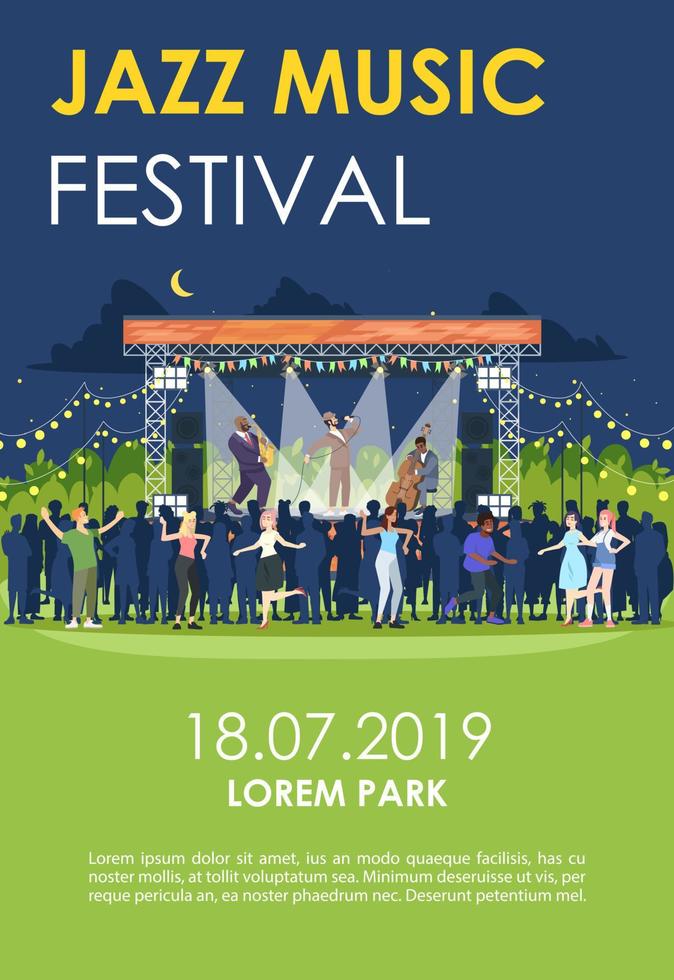This vibrant poster advertises a "Jazz Music Festival" set in Loram Park, dated July 18-20, 2019. The top portion of the poster is predominantly dark blue, with the words "Jazz Music" boldly rendered in yellow against a sky background. Below, "Festival" is written in white, accompanied by a whimsical drawing of a crescent moon and fluffy white clouds. Transitioning to the lower section, the colors shift to a lively lime green, framing the central image of an illuminated stage. Here, three musicians are depicted: a saxophonist in a blue suit, a singer in a brown suit holding a microphone, and a seated cellist. The stage is supported by grey lines and structures, with an enthusiastic audience dancing in the foreground. The overall color scheme includes blue, light blue, green, orange, yellow, purple, and white, reflecting the festive and dynamic atmosphere of a jazz festival.